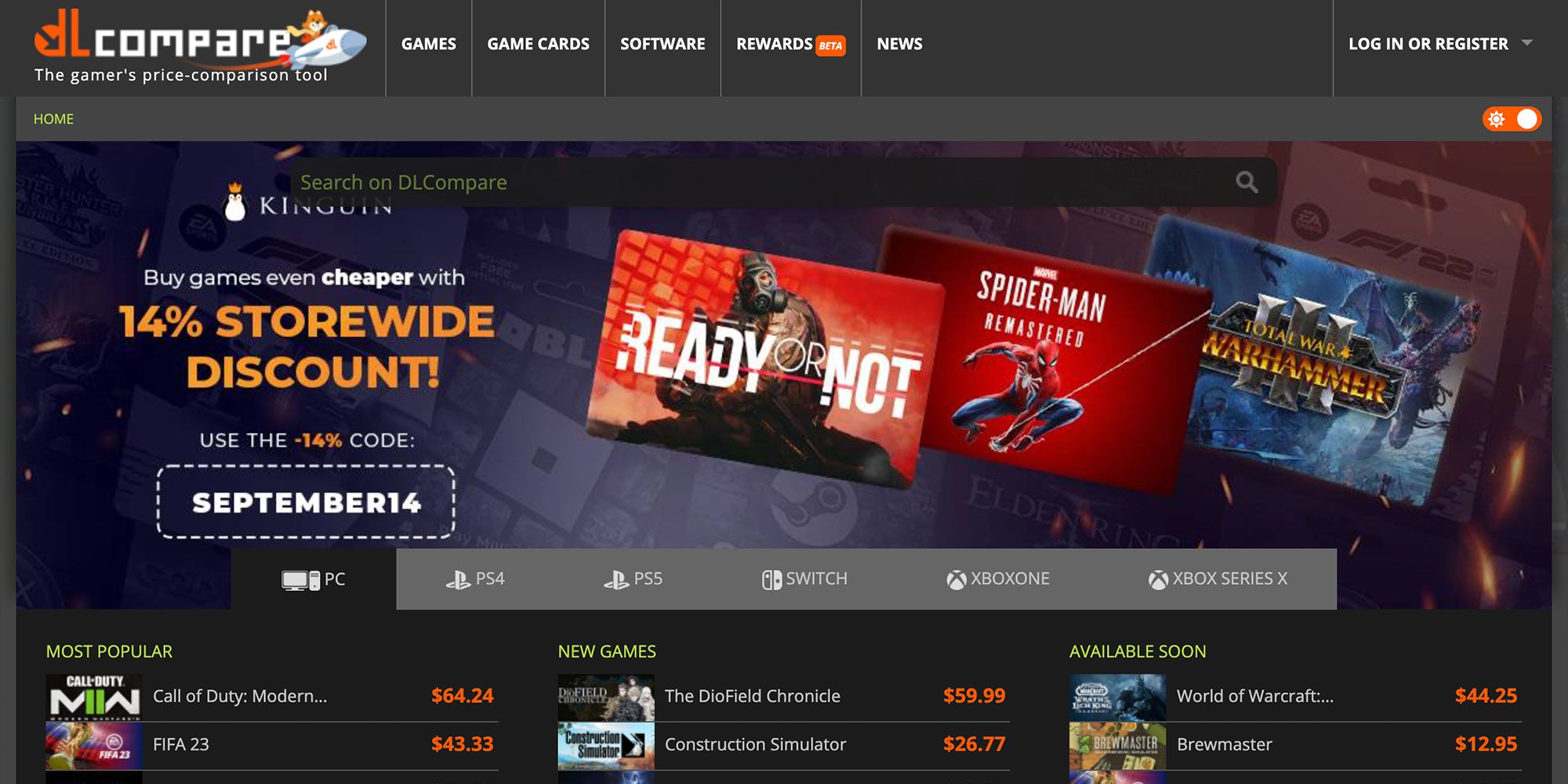Screenshot of the DL Compare Website

The screenshot showcases the homepage of the DL Compare website, with the logo prominently displayed in the top left corner. The logo consists of the letters "DL" in red, "Compare" in white, and a depiction of a fox riding a rocket ship. Adjacent to the logo, the header features a menu bar with several options: Games, Game Cards, Software, Rewards (with a "beta" tag), and News. 

Below the header, a promotional banner occupies the left section of the page, advertising a storewide discount with the message, "Buy games even cheaper with 14% storewide discount." The discount is highlighted in vivid orange text, and the discount code "September 14" is encased in a dashed white line.

In the main content section, images of popular games are displayed, including "Ready or Not," "Spider-Man Remastered," and "Total War: Warhammer." Beneath this, there are lists of games available on multiple gaming platforms such as PS4, PS5, Switch, Xbox One, and Xbox Series X.

The left column features a "Most Popular" section, while the center showcases "New Games." The right column is dedicated to an "Available Soon" section, with prices listed in orange text. Notably, "World of Warcraft" is featured here, priced at $44.25.

In the top right corner of the website, there is a "Login or Register" section for user accounts. Directly below it, an orange toggle button is visible, allowing users to switch between different display settings.